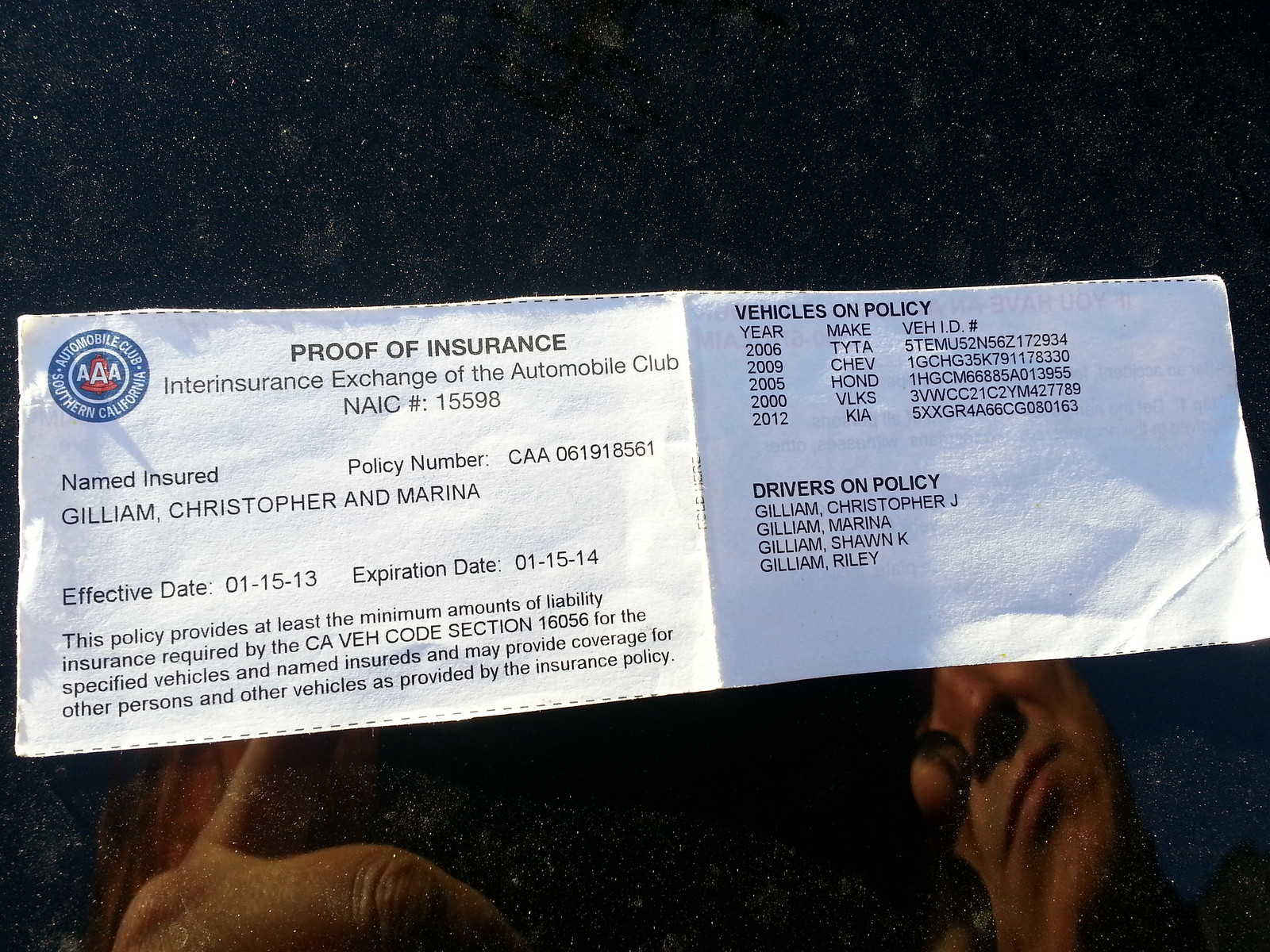In this image, the focal point is a white piece of paper displaying proof of vehicle insurance, likely issued by the Southern California Automobile Club (AAA). The document, folded in half and held up against a reflective surface, probably a dusty black car hood or a window, details insurance coverage provided by the Interinsurance Exchange of the Automobile Club. Key information on the paper includes the NAIC number 15598, policy number CAA 061918561, the names of the insured individuals, Christopher, Marina, Sean K., and Riley Gilliam, and the effective and expiration dates of January 15, 2013, and January 15, 2014, respectively. The paper lists the covered vehicles, including a 2006 Toyota (TYTA), 2009 Chevy, 2005 Honda, 2000 Volkswagen, and 2012 Kia, displaying corresponding vehicle identification numbers. The background of the image features a speckled, almost dirty appearance, possibly due to the reflective nature of the car hood, and faintly shows the reflection of a man's face and hand holding the paper.